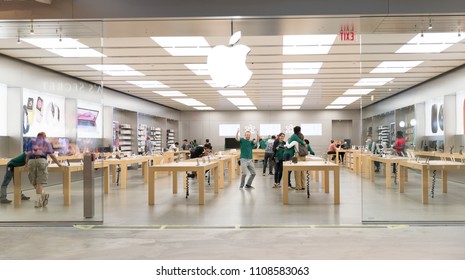This image captures the interior of an Apple Store with its signature modern and sleek design. The store is brightly lit, featuring large glass walls that allow natural light to flood in, creating an open and inviting atmosphere. The centerpiece is the iconic Apple logo prominently displayed. The ceiling showcases a grid of bright rectangular lights that evenly illuminate the entire space. 

The store is spacious and minimalist, consistent with Apple's design ethos. Throughout the store, several large wooden tables are arranged neatly in rows, displaying a variety of Apple products. These tables feature iPhones, iPads, and MacBooks, encouraging customers to interact with the latest technology. Along the left and right walls, shelves and display areas showcase an assortment of products and accessories.

The store is bustling with activity, populated by customers and Apple Store employees, commonly known as "Geniuses," who are easily identifiable by their distinct shirts. Customers can be seen engaging with the displayed products, while others are consulting with employees for assistance. The lively atmosphere underscores the store's role as a hub of technological exploration and customer service.

This image comes from Shutterstock.com, indicated by the watermark at the bottom. The stock image identification number is 1108583063, suggesting that the people in the scene were likely staged for the photo to capture the quintessential Apple Store experience.